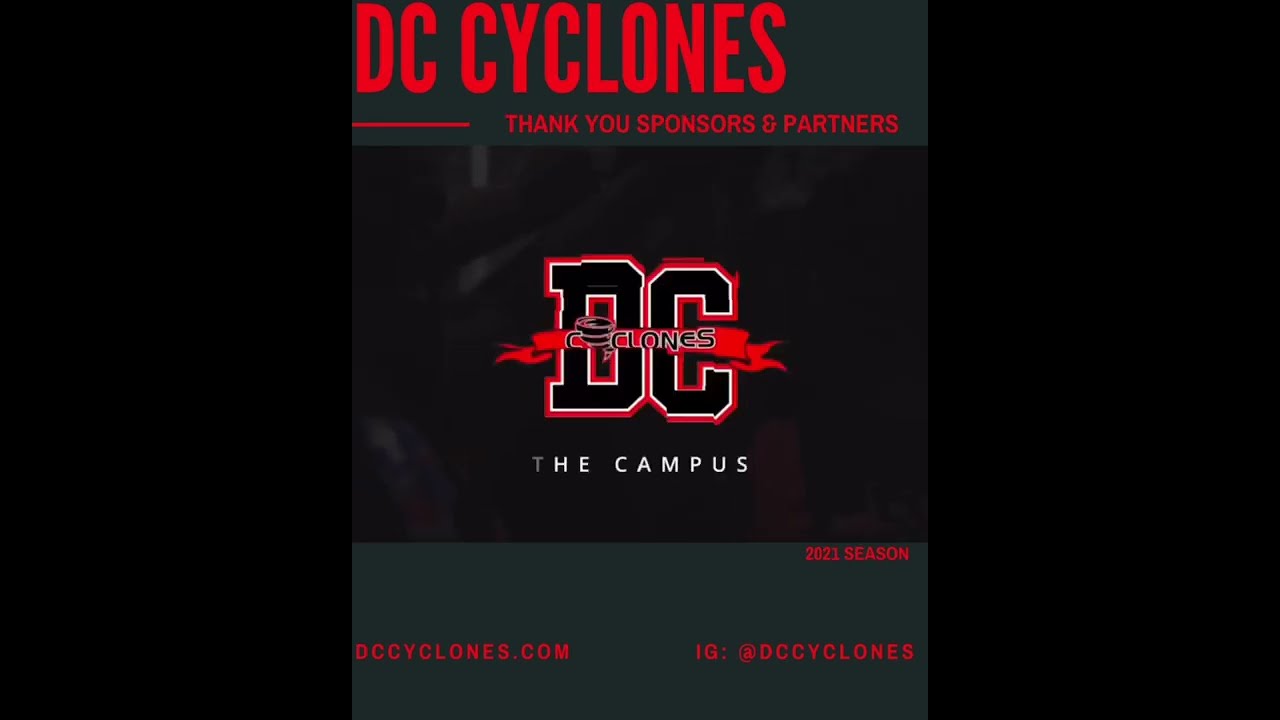The image displays a detailed poster for the DC Cyclones, prominently featuring their appreciation for sponsors and partners. At the top of the poster, “DC Cyclones” is written in bright red text with dark shading, followed by the phrase “thank you sponsors and partners” in the same vibrant style. A red line separates these elements from the rest of the poster. In the center, a large logo showcases “DC Cyclones,” with the letters “DC” in a letterman jacket style and a cyclone symbol replacing the 'Y' in "Cyclones," all set against a sophisticated black marbled background. Below the logo, the words “the campus” appear. Towards the bottom of the poster, additional information is provided in red text, including the 2021 season, the website “dccyclones.com,” and the Instagram handle “@DCCyclones.” The background of the poster includes shades of black and dark green, creating a dynamic and eye-catching design.